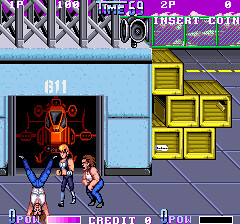The image is a detailed screenshot from a video game scene set in what appears to be an open warehouse or hangar. The background showcases a red-colored aircraft, reminiscent of a helicopter or an airplane. The sky is tinged with a pinkish-purple hue, enhancing the dramatic atmosphere. In the foreground, three men are engaged in a physical confrontation on the bottom left of the image. One man, dressed in a white t-shirt and blue jeans, is performing a handstand, while the other two, also clad in blue jeans and possessing long brown hair, are attacking him. To the right, yellow boxes are scattered around, contributing to the warehouse ambiance.

At the bottom of the image, there is a pinkish bar with the word "POW," accompanied by a black square, and the text “credit zero” is visible as well. Above the scene, game-related text includes "1p" with a score of "100," "time 69" in blue font, "2p" with a score of "0," and “insert coin” displayed in white font. The variety of elements, from the clothing of the characters to the specific on-screen text, provides a rich and engaging depiction of the video game environment.